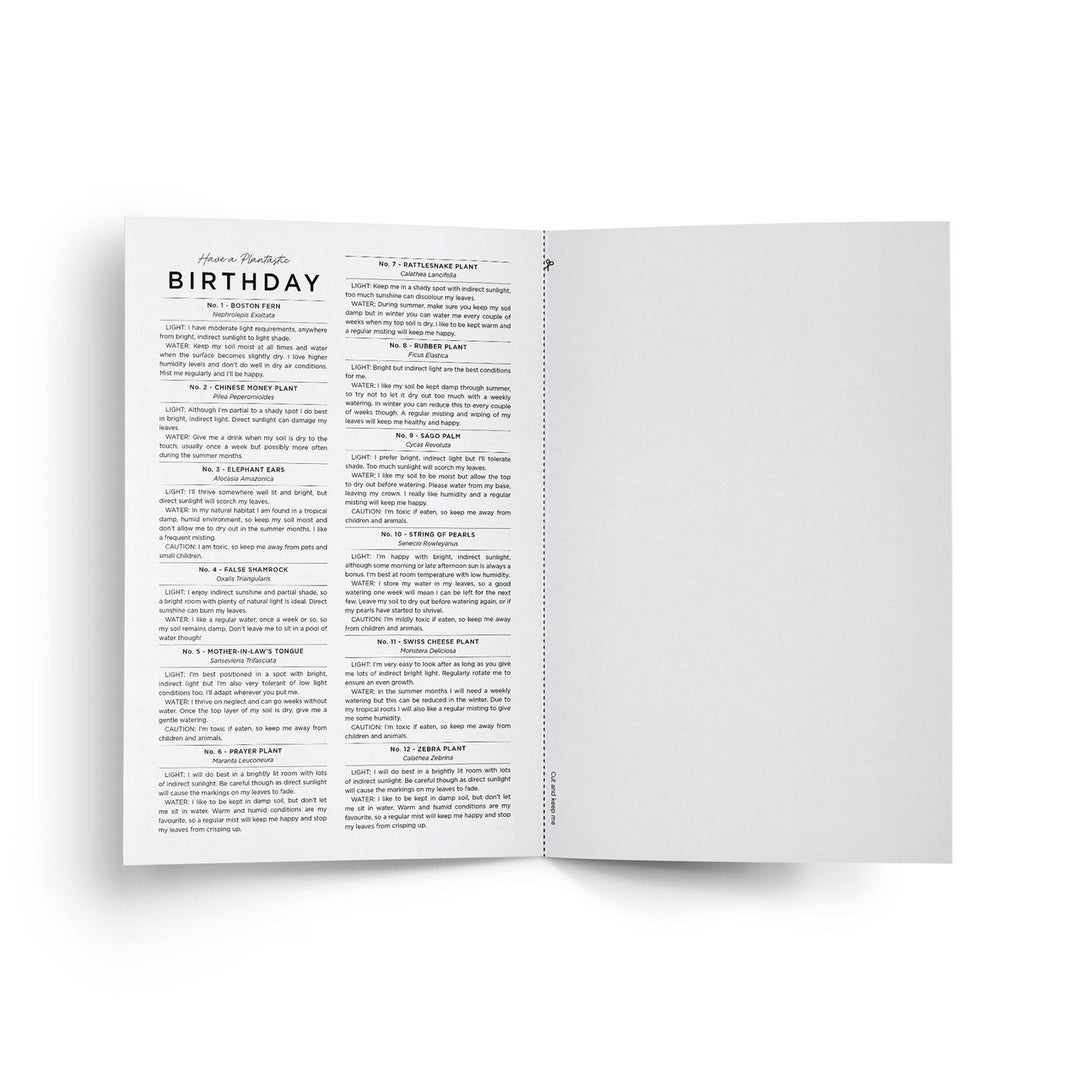The image depicts a foldout card printed on white paper with black text, designed to be cut in half along a dotted line with an illustrated pair of scissors. The left side of the card features an intricate layout: at the top left corner, cursive text reads "Have a plant-tastic birthday." Below this greeting, the card displays a list of plant names organized into two columns, each separated by black lines. The plant names include "busting thread, Chinese money plants, elephant ears, false shamlock, mother-in-law's tongue, prayer plants, rattlesnake plants, rubber plants, sago palm, string of pearls, Swiss cheese plants, and zebra plants." The right side of the card remains blank, underscored by a visual guide for cutting. Despite some blur, the overall impression is that of a monochromatic, well-structured card meant to be an insert or part of a larger document.